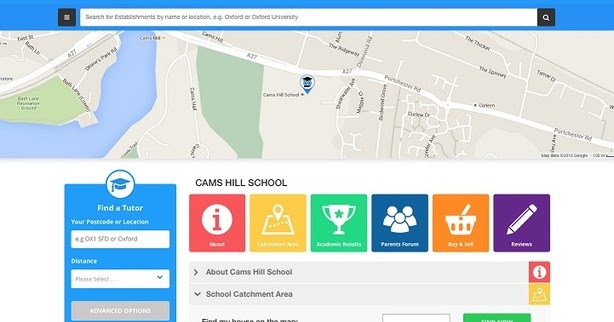Sure, here's a cleaned-up and detailed caption for the image described:

---

The image is a screenshot of a user interface displaying a map. At the top of the screen, there is a blue banner followed by a long, white rectangular search bar. On the left side of the search bar is an icon enclosed in a black square, and on the right side, there is a magnifying glass icon, also in a black square. The search bar contains the placeholder text: "Search for establishments by name or location e.g., Clifford or Clifford University."

Beneath the search bar is a detailed map. Although the map's exact details are not clear due to distance, it prominently displays Cams Hill School marked with a specific icon. 

Below the map, on the left side of the screen, there is a blue box with a graduation cap icon inside a circle and white text that reads, "Find a tutor." This section prompts the user to enter their postcode or location. Beneath it, there is a white search box for user input. Following this, there is text that reads "Distance" in white, accompanied by a drop-down search box, and below that is an "Advanced options" button in a gray box.

Moving over to the right side of the screen, "CAMS HILL SCHOOL" is prominently displayed in black, all-capital letters. Below it are several colored boxes with different functions:
- A red square with an information icon labeled "About"
- A yellow box with a map icon
- A green box featuring a trophy icon
- A blue box that says "Parents Room" with a picture of three people
- An orange box labeled "Buy and Sell" with a shopping cart icon
- A purple box marked "Refuse" with a pencil icon

These sections likely offer additional information and functionalities related to Cams Hill School.

---